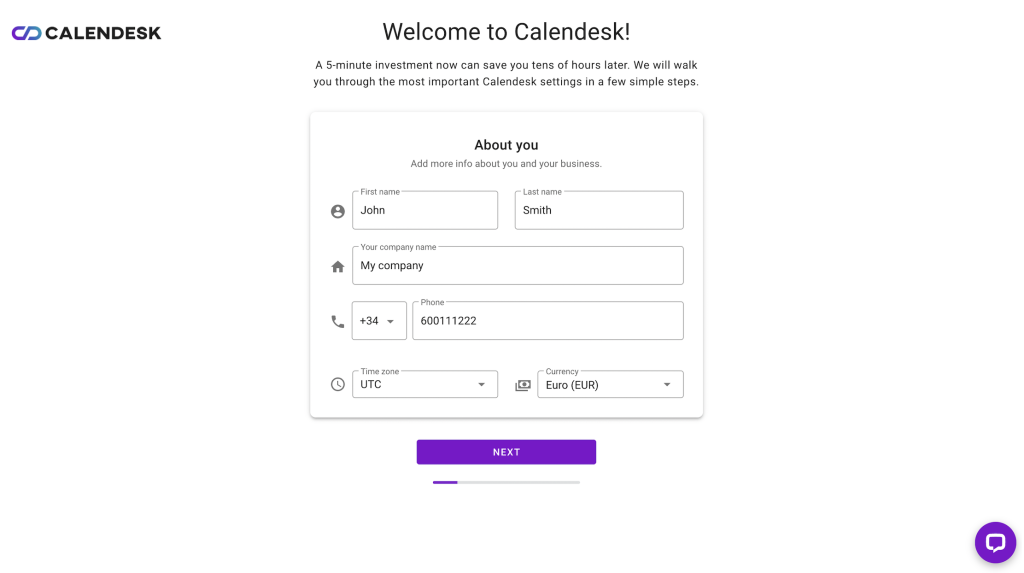The image is a screen capture from the website Calendesk. Positioned at the top left is the text "Calendesk" in black block font, accompanied by a logo to its left resembling a sideways "S" in shades of purple and blue. On the right side of the header, the text "Welcome to Calendesk!" is written in black font. Directly below, a smaller font caption reads: "A five-minute investment now can save you tons of hours later. We will walk you through the most important Calendesk settings in a few simple steps."

The image comprises a square section outlining introductory user details. At the top of this section, the bold title "About You" is displayed, followed by the prompt: "Add more info about you and your business." The first row includes fields for "First Name" with a person icon beside it, pre-filled with the name "John." To the right, the "Last Name" field shows the name "Smith."

The next row contains a section for "Your Company Name," with a small house icon, pre-filled with "My Company." Below this, there's an area for entering a phone number, prefixed by a field for the country code (filled with "+34" and a dropdown arrow) and the phone number "600111222."

Further down, a clock icon precedes the "Time Zone" field, indicated as "UTC" with a dropdown arrow. Next to a money icon, a "Currency" field is shown filled with "Euro (EUR)" and a dropdown arrow for other options.

At the bottom of the square, there's a purple rectangular button with white text that reads "Next." A progress bar beneath this button shows the process is approximately one-eighth completed.